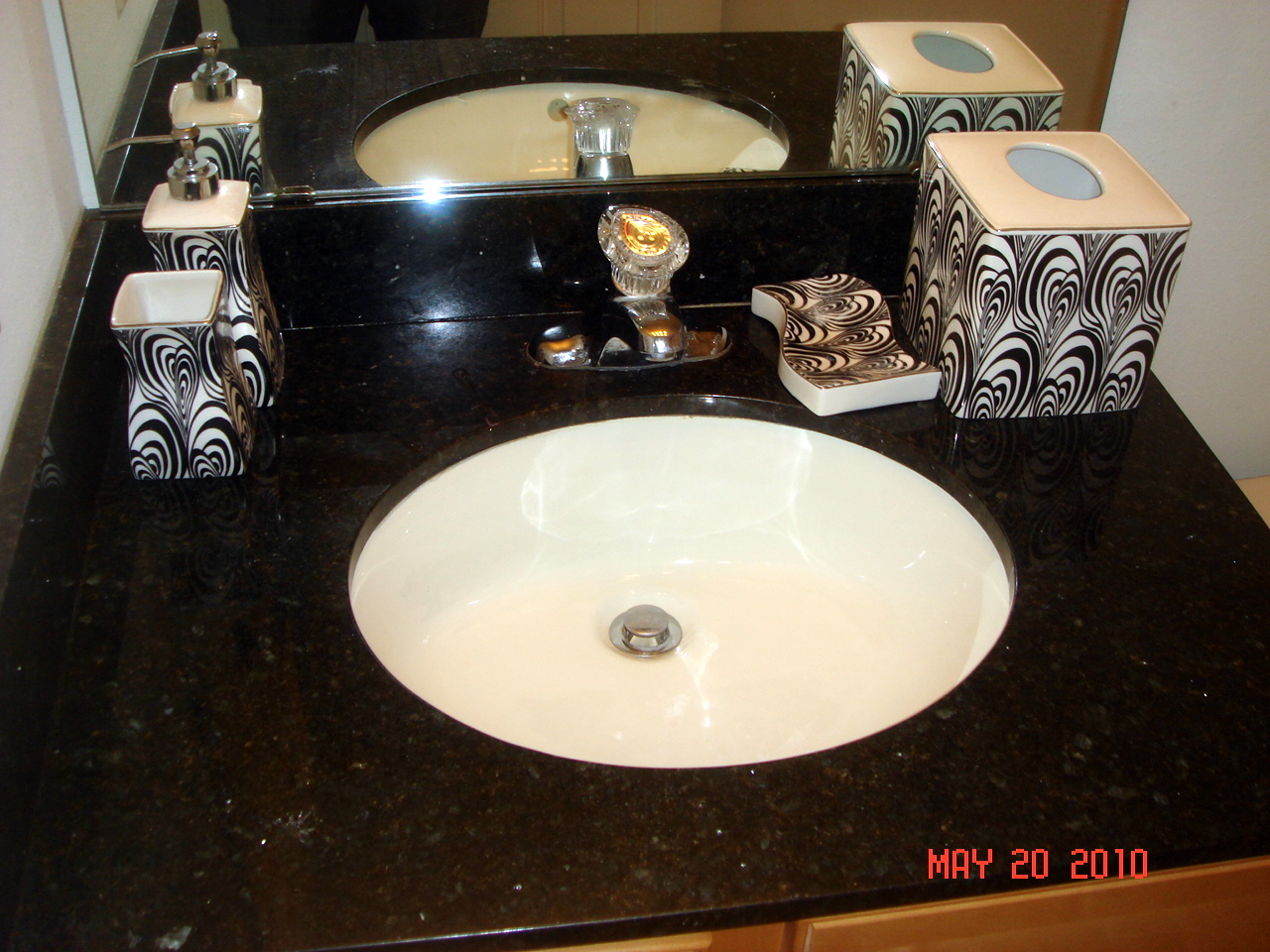This image showcases a neatly arranged bathroom countertop featuring a white sink set against a striking black granite surface. The countertop is partially framed by the visible sections of an orange wooden brown cabinet below. The sink appears round from this perspective, though it could also be oval. A chrome faucet with a single knob is centrally positioned, flanked by a series of coordinated bathroom accessories.

To the left of the sink is a matching black and white swirl-patterned soap dispenser and a small container, creating a cohesive look. On the right side of the faucet, a sponge with the same black and white swirl pattern is neatly placed next to an empty tissue box or cover that sports the same design.

In the background, a strip of the black granite countertop is visible before it meets a mirrored wall. Reflected in the mirror are parts of the faucet's knob, some of the countertop accessories, and portions of the sink and counter. The surrounding walls are painted a clean white, complementing the sleek and modern aesthetic of the space. The photo is dated May 20, 2012, in the bottom corner.